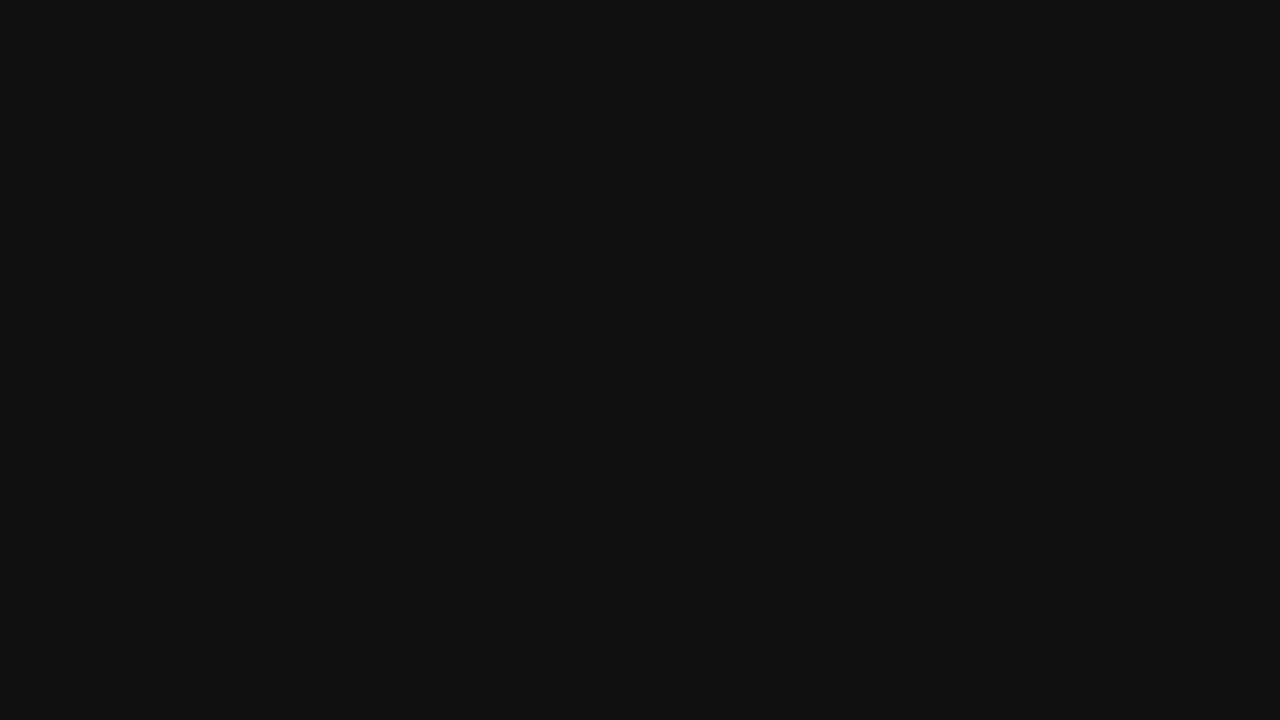This image depicts a completely pitch-black screen, devoid of any visible elements or discernible features. Upon first glance, it appears as an entirely black rectangle, possibly representing a blank laptop or computer screen. There are no objects, figures, or subtle details apparent in the image. Additionally, there is no text or graphical content; if there is any black text, it blends seamlessly with the background and remains invisible. Consequently, changing the text color might reveal hidden messages. The sole characteristic of the image is its unbroken, uniform blackness, offering no insight into what lies beyond this dark facade. There are no children, animals, objects, or items of any sort present in this starkly minimalistic image.